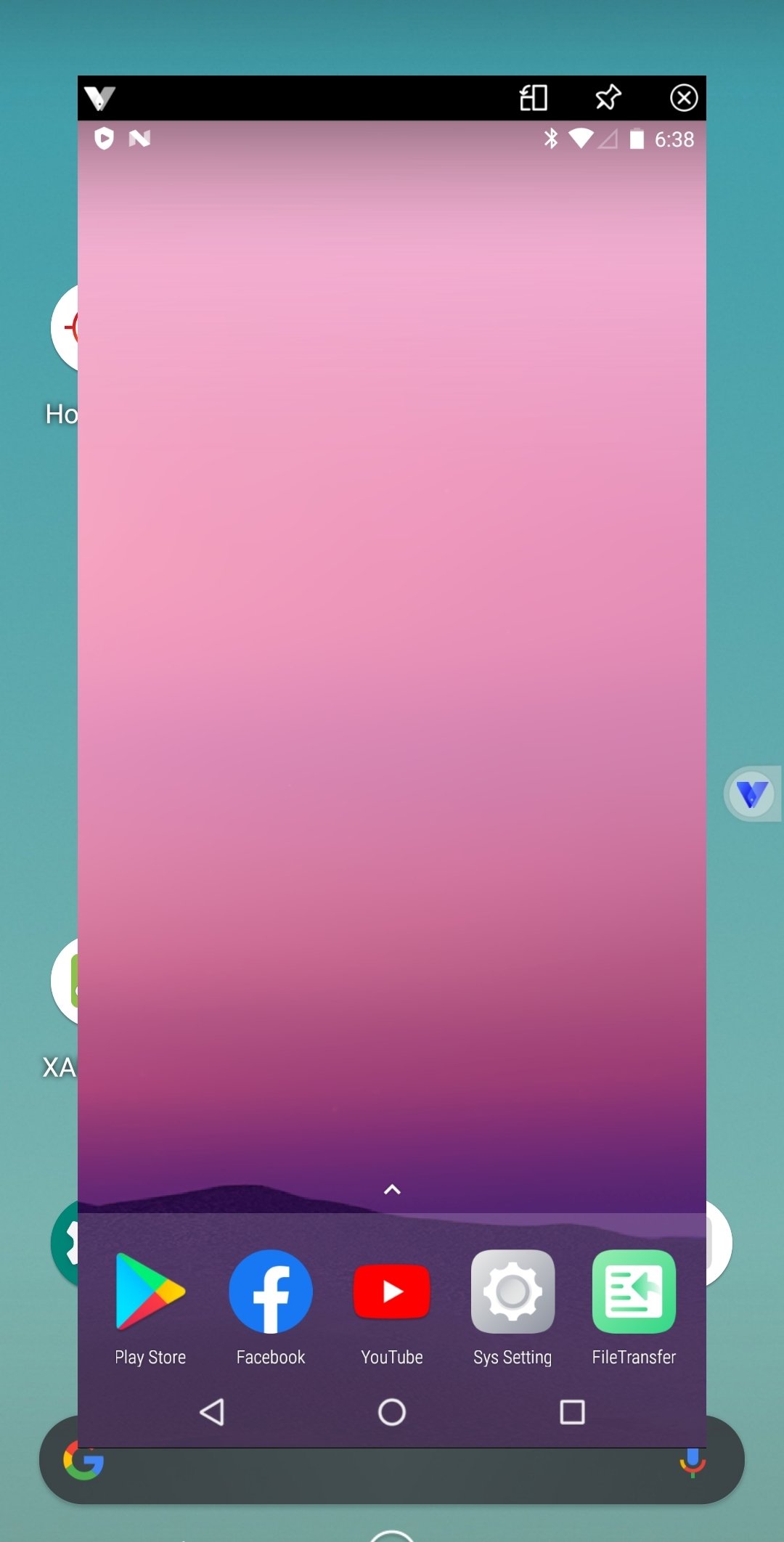The image displays a rich, detailed composition set against a blue gradient background, transitioning to a lighter blue at the center. Prominently featured at the top of the image is a black V-shape with a white left side and gray right side. Below this V-shape, there's a black push pin and a circle containing an X and a rectangle, both resembling app icons or interface elements. 

In the foreground, there is an array of familiar icons: the Bluetooth symbol, the number 638, and a tom (likely referencing a notification badge). The background shifts to a beautiful purple gradient, becoming lightest at the top and darkening towards the bottom where it culminates in a dark purple mountain-like shape. 

At the base of this scene, the purple gradients create an illusion of sand and water, with alternating medium-toned and lighter purple hues. The interface includes several app icons: Play Store, Facebook, YouTube, and a system settings icon labeled "Sys," accompanied by a 'Vowel Transfer' feature.

Towards the bottom of the image, navigation icons are clearly depicted: a left arrow, a circle, and a square, which likely represent the back, home, and recent apps buttons, respectively. Near the base, there is a search bar featuring the multicolored 'G' for Google on the left and a microphone on the right, signifying the ability for voice searches.